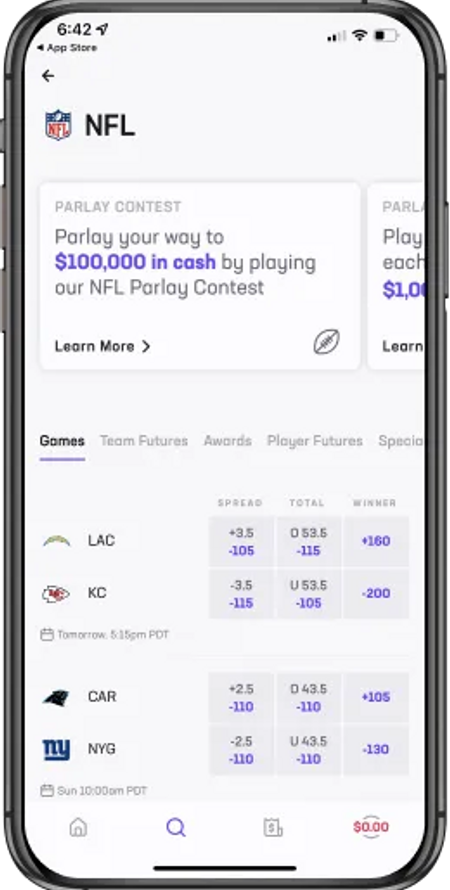Here is the detailed and cleaned-up caption:

---

The image showcases a smartphone screen displaying a sports betting app. The top of the screen indicates the current time, 6:42, alongside icons for sending notifications, Wi-Fi connection, and battery life at approximately 50%. Just below the status bar, there is a back arrow labeled “App Store.” Further down, the app prominently features the NFL logo accompanied by the text “NFL” in black.

The main content area advertises a “Parlay Contest,” allowing users to win up to $100,000 in cash by participating. However, part of the text is cut off on the right side, showing the redundancy of “Parlay Contest.” 

Navigation tabs can be seen below this, labeled as "Games" (currently selected), "Teams," "Team Futures," "Awards," "Player Futures," and another partially obscured tab likely indicating “Specials.” The active “Games” tab lists various NFL matchups, showing teams’ abbreviations, associated spreads, totals, and expected winners.

Highlighted matchups include:
- Los Angeles Chargers (LAC) vs. Kansas City Chiefs (KC), with respective spreads, totals, and winners listed.
- Carolina Panthers (CAR) vs. an unspecified team, notated similarly.
- New York Giants (NYG) vs. an unspecified team, notated similarly.

A calendar icon denotes game times, such as “Tomorrow at 5:15 PM PDT” and “Sunday at 10 AM PDT.”

The bottom border of the screen includes navigation buttons: a home icon, a search icon, a money bag icon, and an indicator for account balance showing $0.00.

---

This enhanced caption provides a clear and comprehensive description of the smartphone screen content, making it easier for readers to visualize and understand the context.